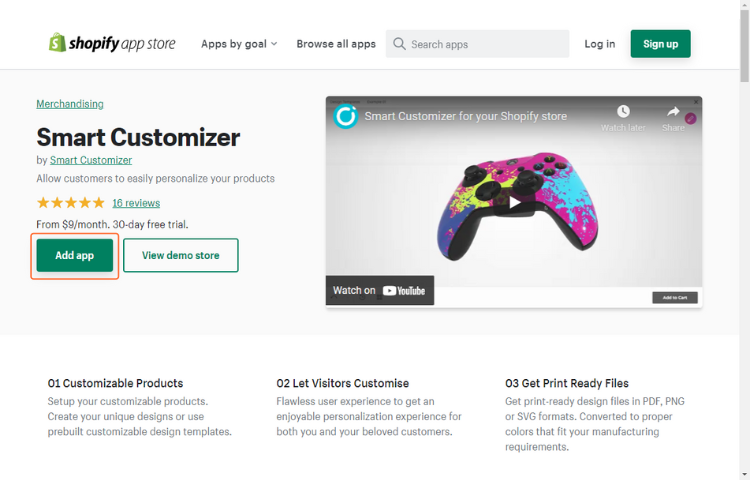The image showcases the Shopify App Store interface, with the distinct Shopify logo—a green shopping bag adorned with a dollar sign—prominently displayed in the top left corner. The navigation bar features a drop-down menu labeled "App by Goal," accompanied by options to "Browse All Apps." To the right of the menu, a gray search bar is positioned, inviting users to "Search Apps."

Adjacent to the search bar, there are two buttons: a standard "Log In" button and a prominent green "Sign Up" button. Below this section, the interface transitions to a light gray background highlighting a featured app under the "Merchandising" category. The app, "Smart Customizer by Smart Customizer," boasts a 5-star rating garnered from 16 reviews and offers pricing starting at $9 per month with a 30-day free trial.

To the right of this pricing information, a green "Add App" button, outlined conspicuously with a red box, is positioned for user interaction. Below it, a white button with green text prompts users to "View Demo Store." Adjacent to these buttons is an embedded YouTube video, titled "Smart Customizer for your Shopify store." The video thumbnail features a colorful game controller in shades of purple, yellow, and blue, indicating a visual example of the customizer's capabilities.